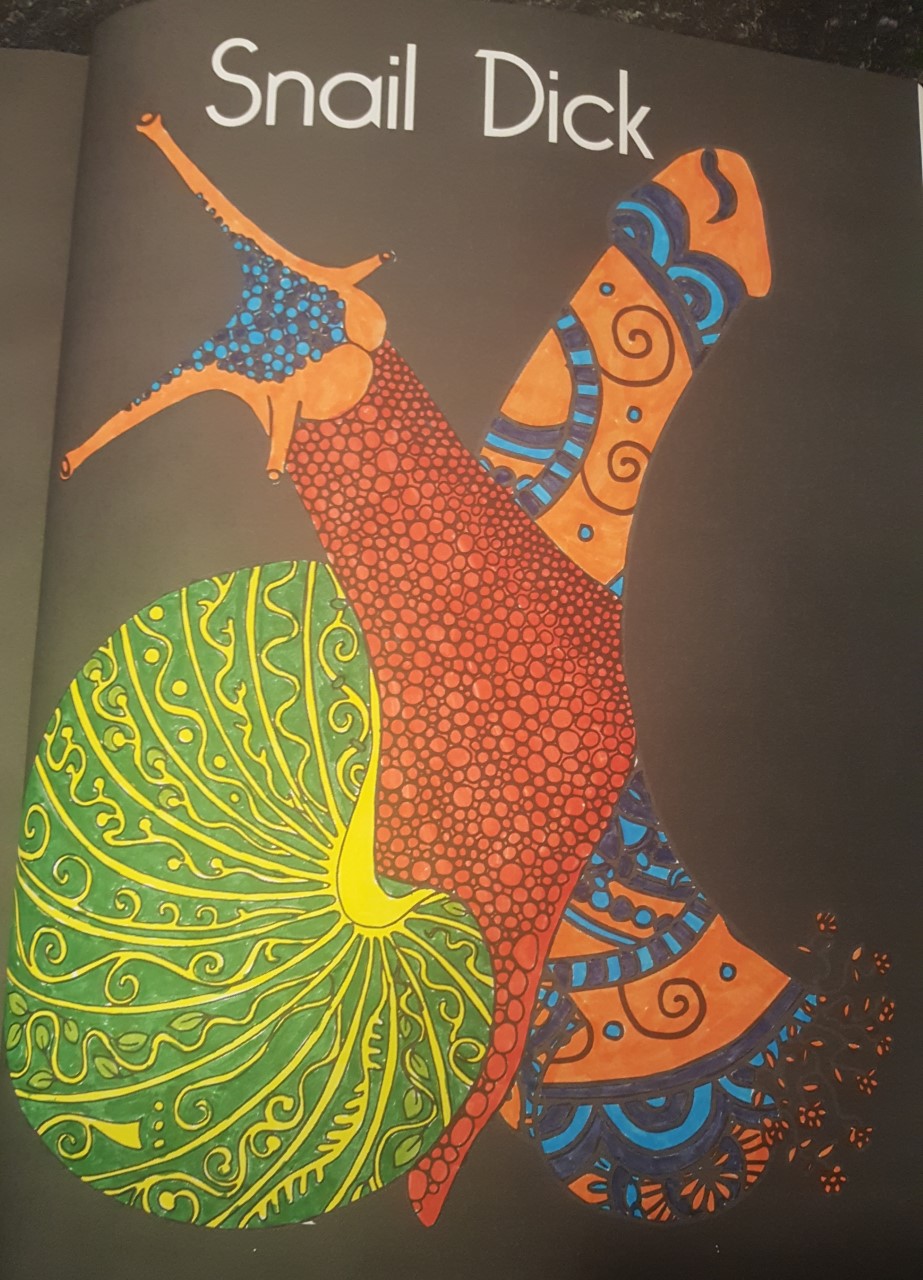This is a vertically framed image depicting a page from a book, specifically the right page. The page has a brownish hue, contributing to a vintage or aged appearance. At the top of the page, in bold white lettering, the title "Snail Dick" is prominently displayed. Below the title is an intriguing piece of artwork. 

The artwork features a large snail shell, rendered in green with white lettering and wavy lines creating a textured effect. The body of the snail occupies the center of the image, extending upward and slightly to the left. It is colored a vibrant red and is covered with interconnected dark circles, lending it a unique, almost mosaic-like texture. The head of the snail, outlined in orange, displays a striking contrast with a blue top speckled with black circles. 

Additionally, emerging from the lower right corner of the frame and curving upward towards the upper right is the form of a penis. This part of the image features a primarily orange color scheme, accentuated with stripes and curves in varying shades of dark and light blue, adding a dynamic and somewhat surreal element to the composition.